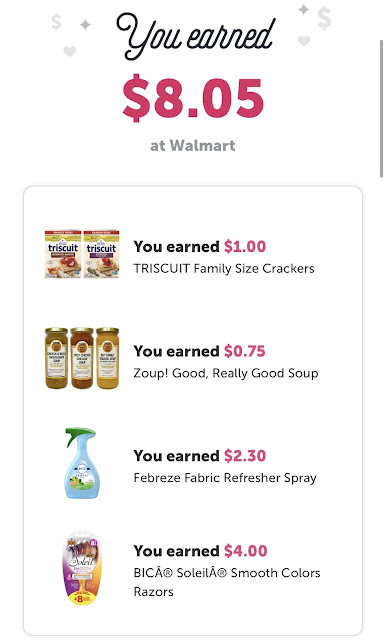**Descriptive Caption:**

The image is a screenshot taken from a phone, showcasing a rewards summary from a cashback or rebate app. At the top of the screen, there are icons for a dollar sign, a heart, and a diamond on both the upper left and right corners. The header reads, "You earned $8.05 at Walmart," highlighting a total cashback amount of $8.05. 

On the right side of the screen, a scroll bar indicates that more rewards can be viewed by scrolling down. The main content of the screenshot displays several transactions:

1. **Triscuit Family-Sized Crackers:** An image of two boxes of Triscuits accompanied by the text, "You earned $1.00 Triscuit family-sized crackers."
2. **Soup:** An image of three jars of soup with the caption, "You earned $0.75, soup, good, really good soup."
3. **Febreze Fabric Refresher Spray:** An image of a bottle of Febreze Fabric Refresher Spray, stating "You earned $2.30, Febreze Fabric Refresher Spray."
4. **Bic Soleil Smooth Colors Razors:** A picture of a package of razors with the note, "You earned $4.00 from Bic-A, Soleil-A, Smooth Colors Razors."

This screenshot likely comes from a cashback app similar to Ibotta, which rewards users for purchasing specific items at participating retailers.